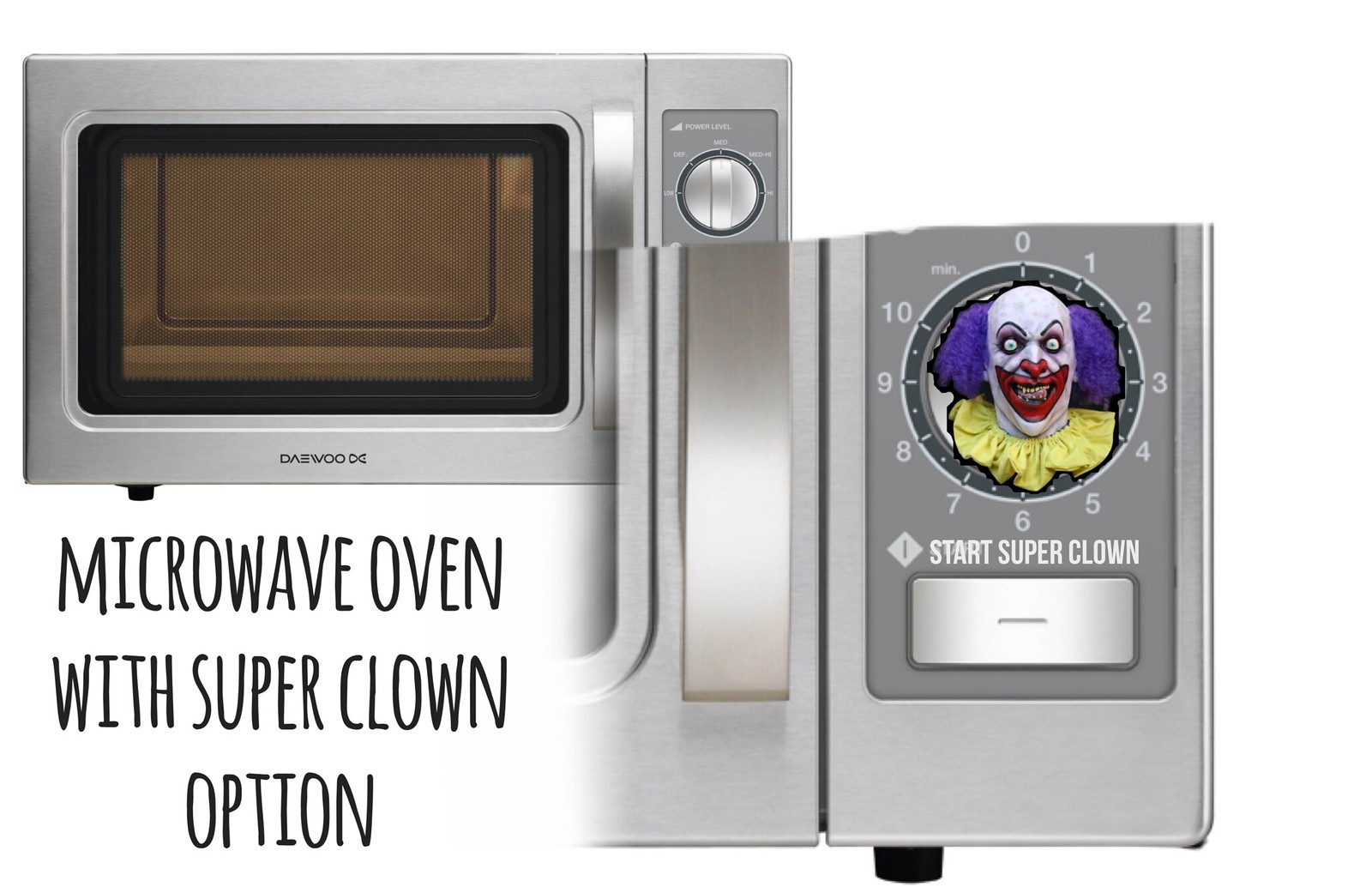The image is a composite of two photographs arranged in a rectangular landscape layout. The left part of the image shows a traditional silver microwave oven with the brand name "Daywood" visible. The microwave appears empty with a wind-up dial on the top and a visible pop-open button at the bottom. Below the microwave, there is black text stating "Microwave oven with super clown option." The right part of the image features a close-up of the microwave's bottom right corner, specifically highlighting the dial and start button. The dial is numbered from 0 to 10 and prominently displays an image of an ominous-looking clown with big red lips, poofy purple hair, and a yellow ruffle collar in its center. Below the dial, a rectangular button reads "start super clown." The overall absurdity of combining a microwave oven with a "super clown option" suggests the image may be a joke or parody.